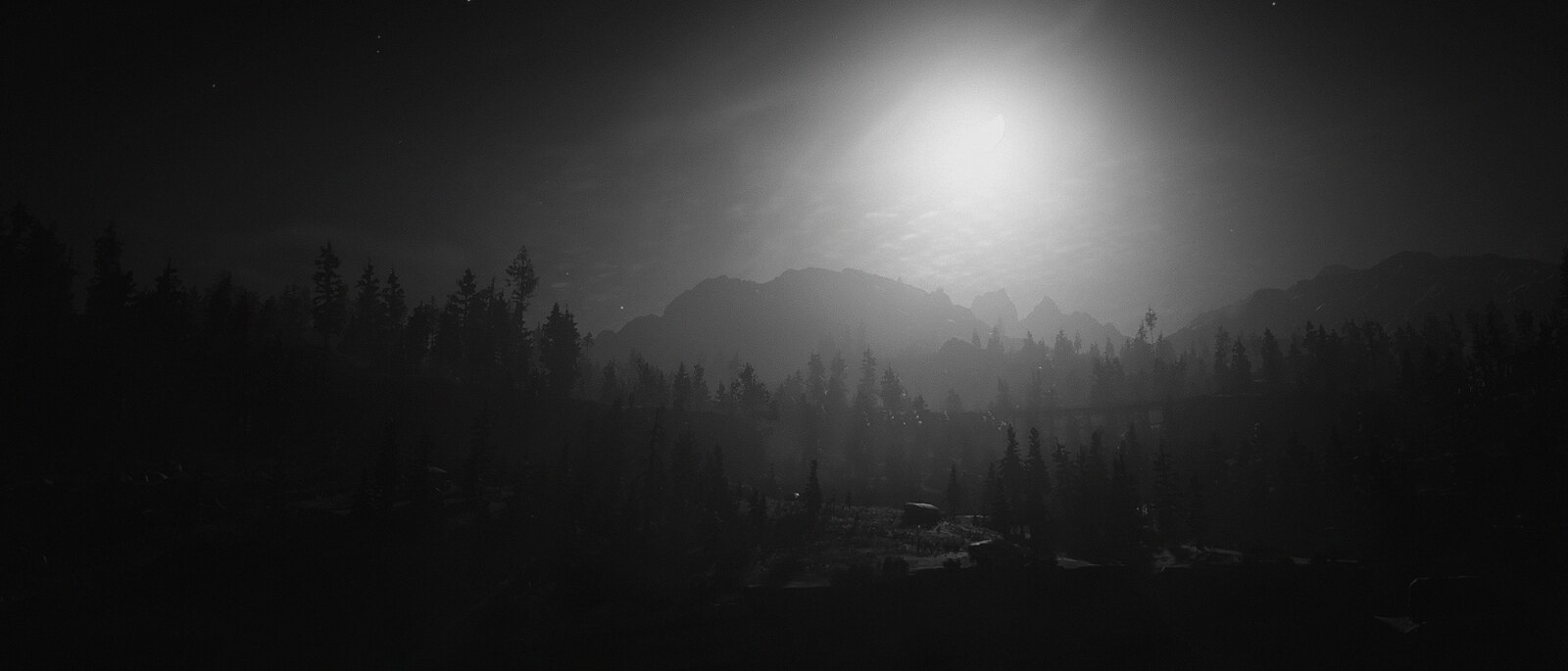This is a sepia-toned black and white landscape image taken with a very wide angle, roughly three times as wide as it is tall. The central upper part of the image features a bright light source, likely the moon, sitting slightly to the right of center, which casts a glow through the cloud layer. Below this light source, the rugged silhouette of mountainous terrain is visible, bearing a distinct ridge that gives it character. The foreground is dominated by the dark silhouettes of hundreds of fir-like pine trees, creating a secluded, dense forest appearance. The color palette ranges from near-black at the bottom of the image through various shades of dark grey and brown as it ascends, emphasizing the depth and expanse of the landscape. The sides of the image are enveloped in near-total darkness, drawing the viewer's focus to the illuminated middle section, making the contours of the mountains and trees stand out starkly against the lighter sky.